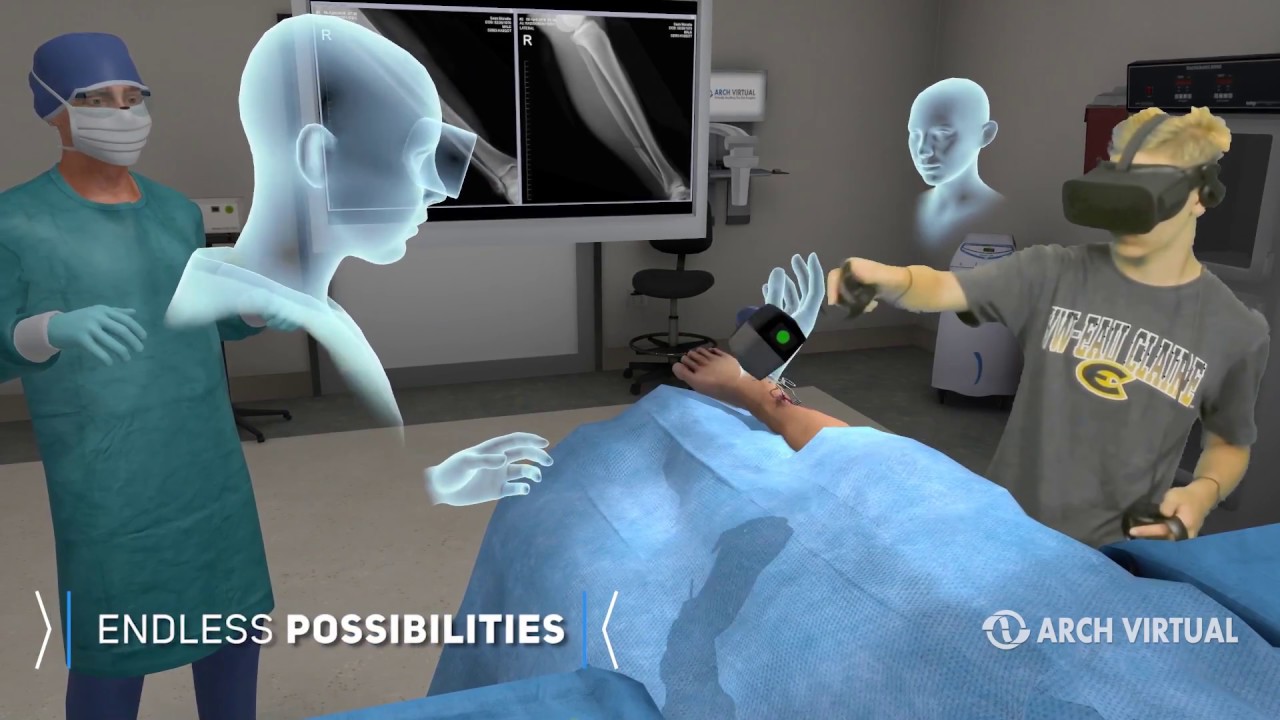The digital image depicts a virtual reality simulation of a medical procedure set in an operating theater. On the left, a healthcare professional, possibly a doctor or nurse, stands to the side wearing a surgical mask and gloves. On the right, a young man with blonde hair is engaged in the simulation using a VR headset and controllers, seemingly conducting a procedure on a patient who lies on the table covered in a blue sheet. Ghostly digital figures, representing additional virtual participants, flank both sides of the scene. An x-ray image of the patient's leg is displayed on a monitor in the background. Text on the image includes "endless possibilities" in the bottom left corner and "Arch Virtual" on the bottom right, highlighting the potential applications of virtual reality in medical settings.